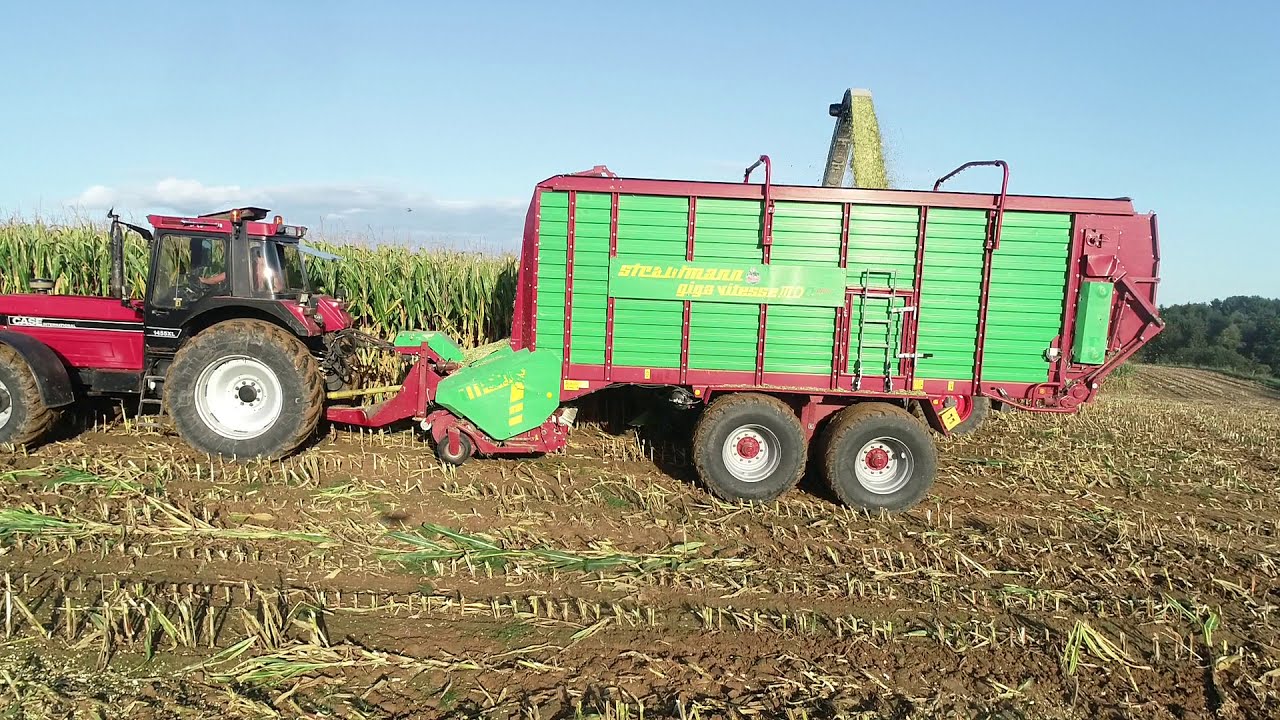In this color photograph taken from a slightly elevated vantage point, possibly by a drone, you can see a red tractor with a green and red trailer in a vast cornfield. The foreground shows the remnants of previously harvested corn with muddy terrain and stubby stalks, indicating recent plowing activity. The tractor, facing left, is located about halfway up on the left side of the image. It is apparent that the tractor is in the process of harvesting, as it tows a large cart designed for collecting grain. The trailer, featuring stacks of green items arranged in multiple rows, has a visible nozzle or conveyor mechanism actively shooting grain into its back. Behind the tractor, the field is populated with tall, standing corn, while further in the background, you can spot additional plowed cornfields, a mountainous area, and a light blue sky graced with a few clouds near the horizon. The scene captures the essence of agricultural work amidst a picturesque landscape, blending the raw elements of farming with the serenity of nature.